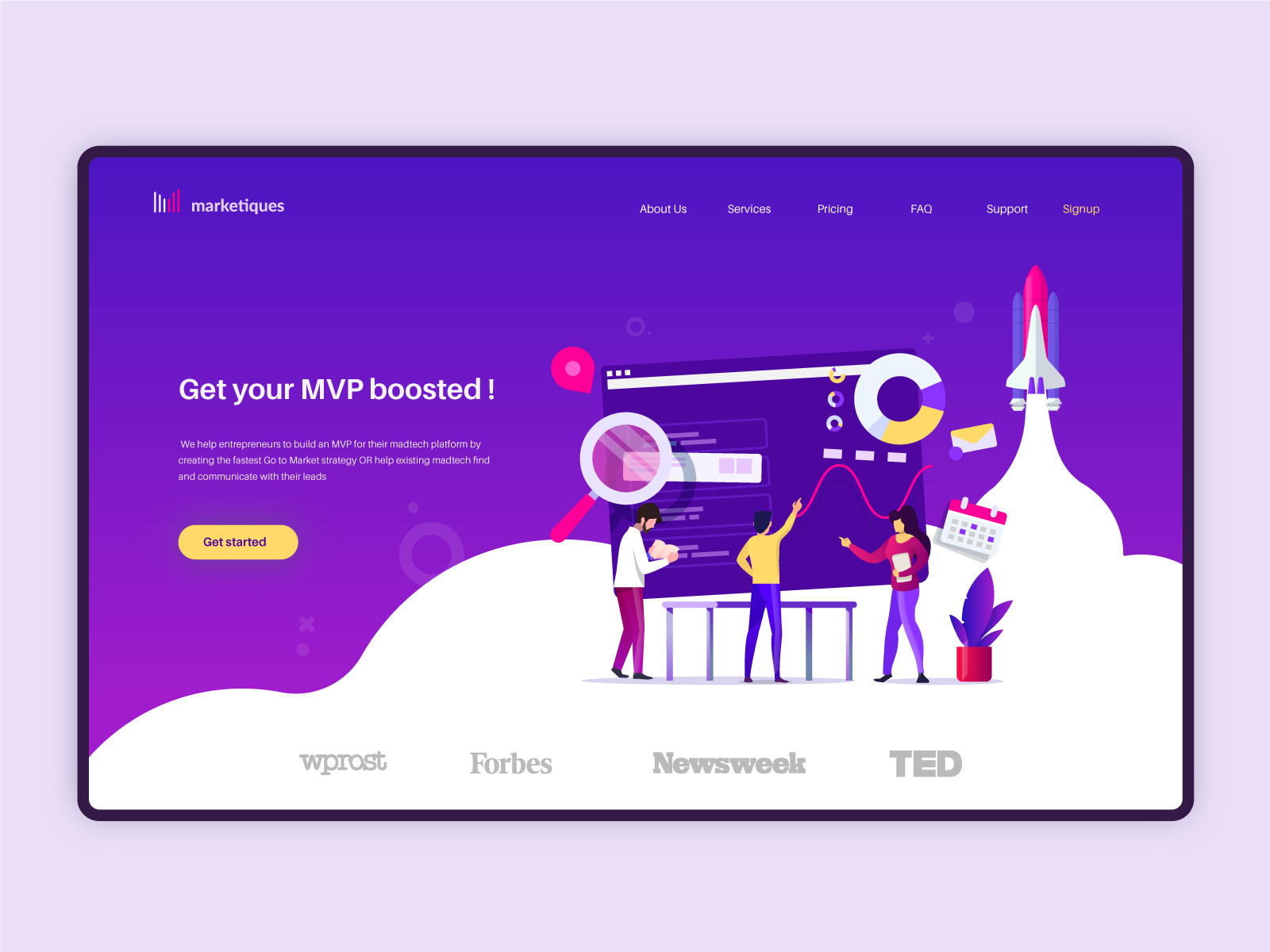This is a detailed screenshot of a website named Market Teaks. The background is bright purple with a wavy white section at the bottom, reminiscent of snowbanks. From the white area on the right, a rocket is depicted launching vertically towards the upper right corner of the page. The rocket features a pink base, white body, and two blue segments on its sides.

Dominating the center of the page, slightly to the left, is a large dark purple rectangle that closely resembles a chalkboard with a white horizontal line across the top. This "chalkboard" serves as a focal point and may simulate a drawing or presentation board. In front of it, there are illustrations of three people—two men and one woman—engaged in what appears to be a discussion or presentation.

At the bottom of the page, the text "W. Prost, Forbes, Newsweek, and TED" is prominently displayed, likely indicating affiliations or endorsements. To the center-left of the image, bold white text reads, "Get your MVP boosted. We help entrepreneurs build an MVP for their mad tech platform by creating the fastest go-to-market strategy or help existing mad tech find and communicate with their leads."

This descriptive caption ensures the reader has a clear and vivid understanding of the webpage's visual elements and messaging.